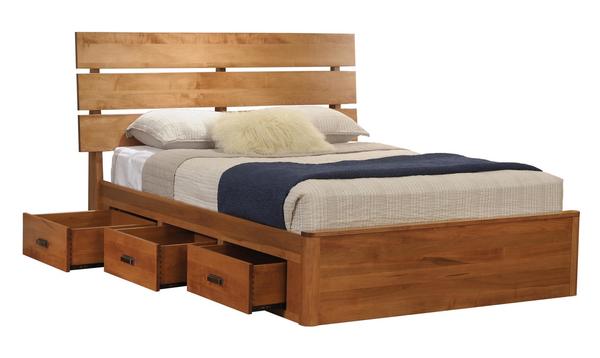The photograph showcases a stylish, medium brown wooden framed bed with a distinctly Scandinavian design reminiscent of Swedish furniture from IKEA. Its headboard is composed of three horizontal slatted boards with slight gaps in between, adding a touch of visual interest. The bed features three drawers along the left-hand side, each progressively pulled out to varying extents to demonstrate their storage capacity; the drawers are brown with dark brown standard handles. The mattress, likely a full-size, is thin and topped with a neatly tucked blanket featuring tan burlap with blue and tan stripes. There are three pillows adorning the bed: two flat white ones and a fluffier, cream-colored fur pillow. The backdrop is a plain white wall, and the bed exudes a clean, minimalist aesthetic.